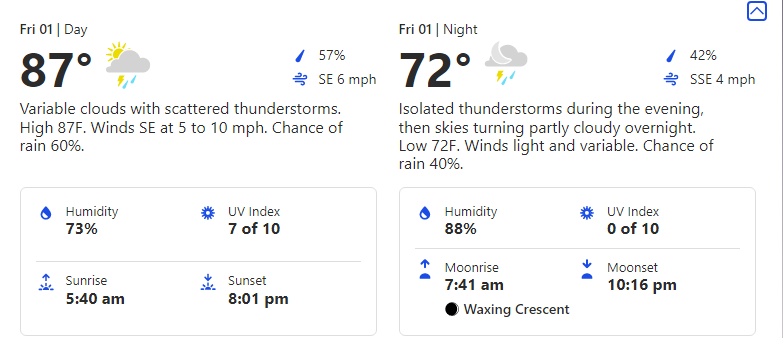In the image, a detailed weather forecast is presented. In the top left corner, the title indicates it's for "Friday 01." The current temperature is shown to be 7 degrees Fahrenheit with a description of variable clouds and scattered thunderstorms expected. The high temperature for the day is 7 degrees Fahrenheit. A southeast wind is blowing at speeds ranging between 5 to 10 mph. There's a 60% chance of rain with a humidity level at 57%.

Additional weather details include the wind speed precisely measured at 6 mph coming from the southeast, and a UV index rated 7 out of 10. The sunrise is scheduled for 5:40 a.m., while sunset is expected at 8:01 p.m. Moving to "Friday 09," the temperature climbs to 72 degrees Fahrenheit. The evening is predicted to have isolated thunderstorms, with the sky gradually becoming partly cloudy. A closing note thanks viewers for watching.